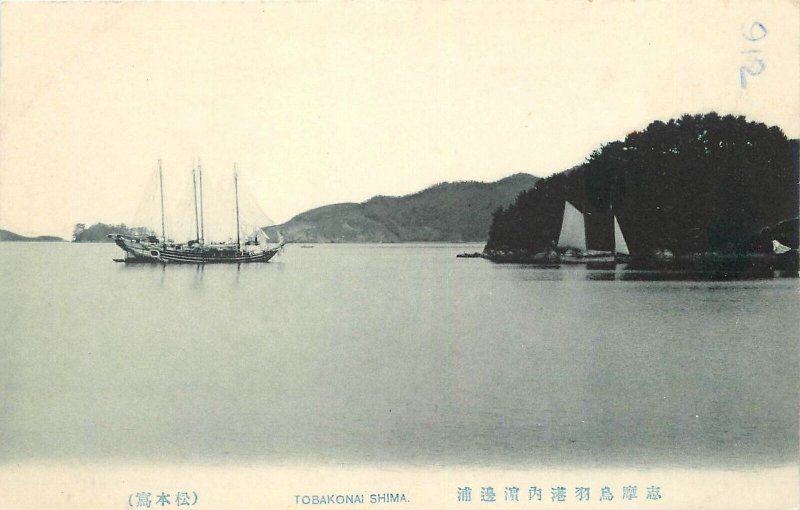The photograph is a vintage, slightly faded black-and-white image with a bluish hue, possibly due to age. It depicts a tranquil body of water, which appears still with only a slight ripple. This body of water could be a lake or the ocean. In the scene, there is a long fishing boat with four masts and translucent sails, floating elegantly on the water. This boat, resembling an Asian junker-style vessel, is positioned near the center. To its right, there's a smaller sailboat. Both vessels seem anchored near a modestly sized island covered mainly in lush, bushy trees.

In the background, there is another larger landform, potentially another island or a part of the mainland, also covered in vegetation. The sky above the scene is featureless and stark white due to the black-and-white nature of the photograph.

Written in blue pen in the upper right corner of the photograph, oriented sideways, is the number "912." At the bottom of the image, there is a text in a mix of white-blue font and Japanese characters, stating "Tobakonai Shima," which could be a name or location. Additional Japanese lettering is adjacent to this text. The photograph has the appearance of being on or part of a card, with the surrounding area of the card having a yellow, faded coloring, possibly enhancing the vintage feel of the image.